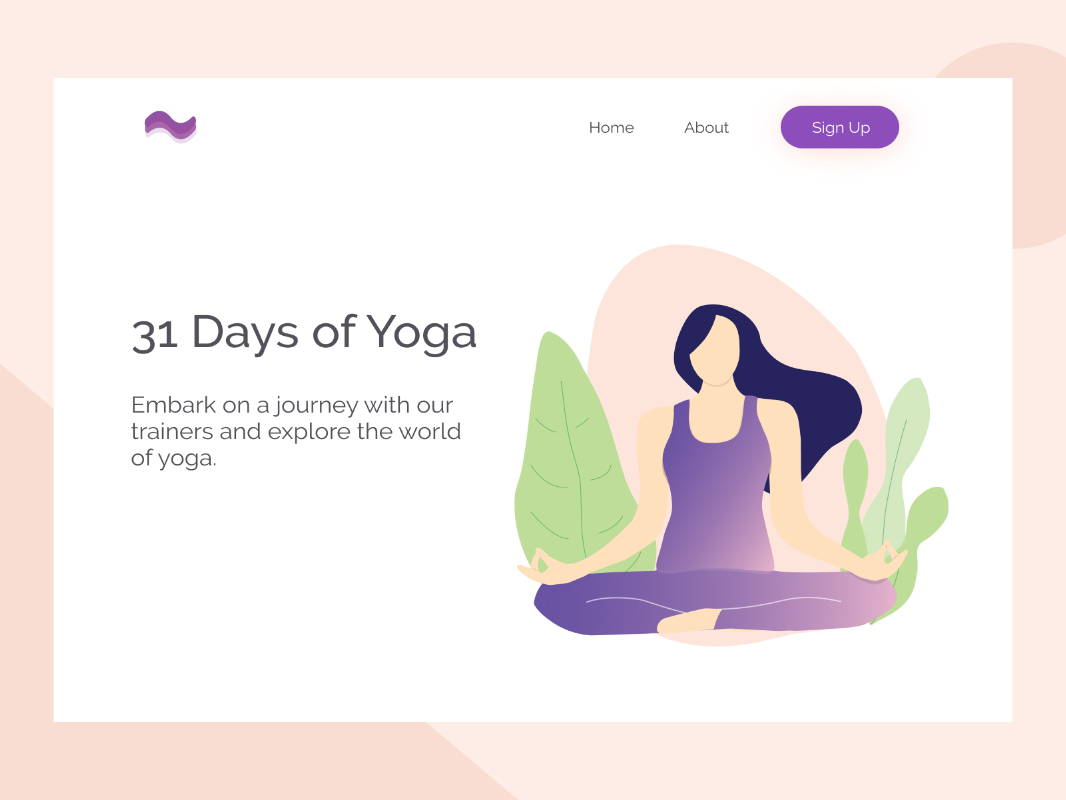The image showcases a promotional graphic for a 31-day yoga program. At the center, a woman with long black flowing hair is depicted in a yoga pose, seated cross-legged with her wrists resting on her knees, and her index fingers and thumbs touching. She is dressed in a purple tank top and matching purple pants. Above her, on a white background framed by a rose gold border, are the words "31 Days of Yoga" in prominent text, and below it in smaller, unbolded text, it reads: "Embark on a journey with our trainers and explore the world of yoga."

In the upper portion of the graphic, flanked by a picture of a large leaf and a cactus on one side, are the website navigation options labeled "Home," "About," and "Sign Up" in purple buttons, separated by a wavy purple line. The top right corner features an artistic depiction of a sun in varying shades of rose gold and orange. The entire graphic is designed with a clean, welcoming aesthetic to encourage potential participants to join the yoga program.